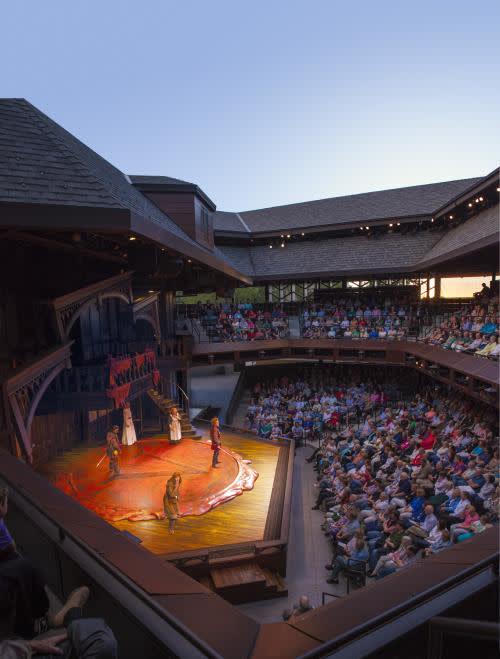This photograph captures a vibrant scene at an outdoor amphitheater during what appears to be sunset, giving the background a warm, orange glow. The amphitheater features tiered wooden seating in mid-tone chocolate hues with white accents, and it is filled with a diverse audience dressed in an array of colors and styles including shades of blue, red, tan, green, pink, orange, white, and yellow. The focal point of the image is the stage, where performers clad in medieval-inspired costumes are engaged in what seems to be a theatrical performance. Among them are both men and women, with outfits ranging from flowing white dresses to a shorter green dress. One man is notably holding a sword. Above the stage is a wooden balcony, adding an architectural detail, and a staircase is visible beside one of the women in a white dress, enhancing the depth and setting of the scene.